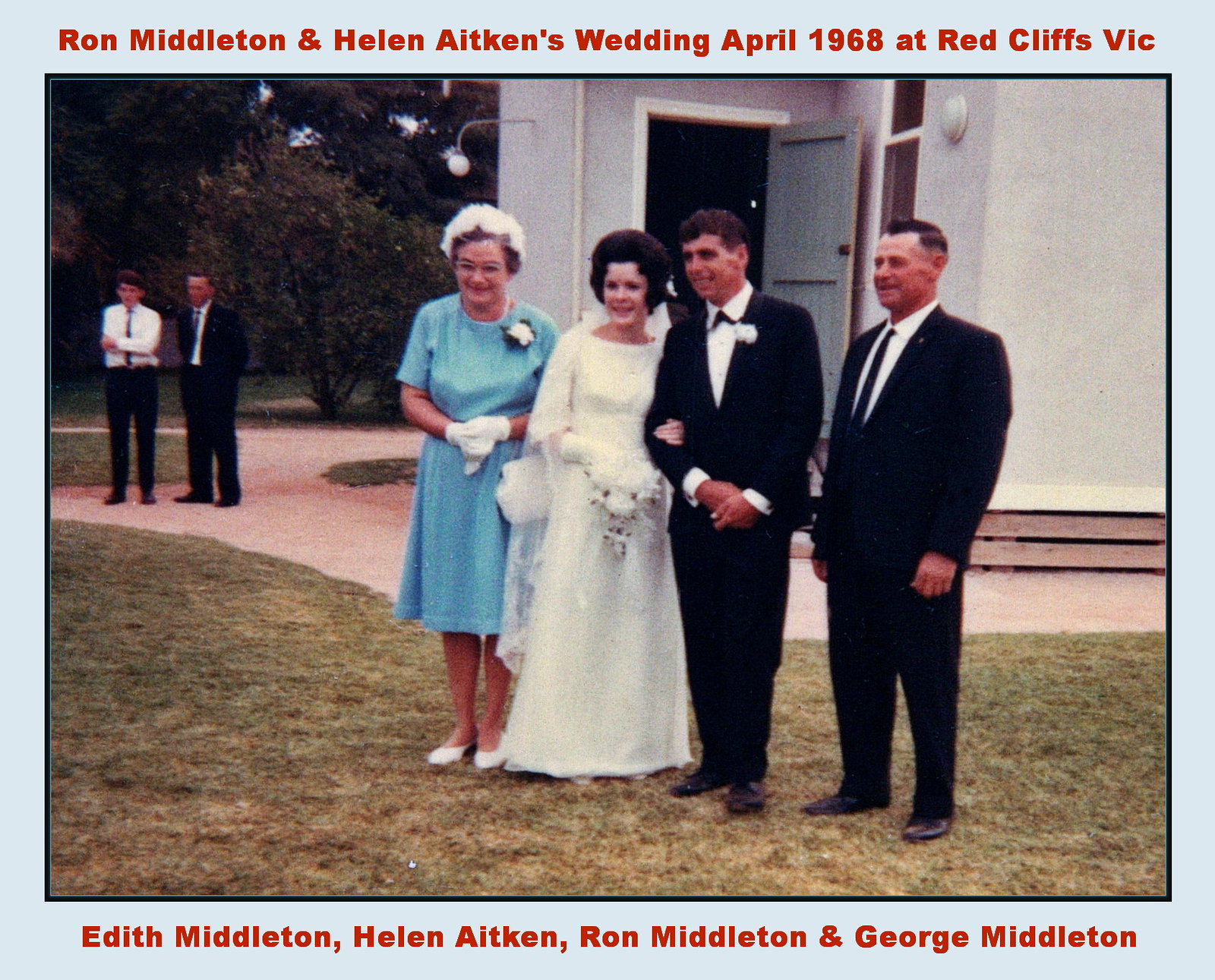The photograph captures a vintage wedding scene from April 1968 at Red Cliffs, Vic, framed with a light blue border. In the foreground, four individuals pose in front of what appears to be a church or community center with a blue wooden door adorned with exterior lights. On the left, Edith Middleton stands elegantly in a blue dress, white gloves, and a white hat, with a white flower pinned to her attire, signifying her role as the mother of the bride. Beside her is the bride, Helen Aitken, donning a classic white wedding dress and black hair. Holding Helen's arm is the groom, Ron Middleton, dressed in a tuxedo with a white shirt. On the far right, George Middleton, likely the father of the groom or bride, is seen in a black suit with a white shirt and black tie. They are positioned on a green lawn, which shows patches of wear, with a dirt path visible behind them. In the distance to the left, two men dressed in business attire, possibly wedding attendees, engage in conversation on a sidewalk. The photograph is captioned in red lettering with their names: Edith Middleton, Helen Aitken, Ron Middleton, and George Middleton.